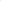The image is a completely blank white space without any objects or colors. However, there is a prominent yellow box outlined in a deeper yellow border. Inside this box, various prompts guide the viewer to consider potential elements within an imaginary image. At the top of the yellow box, a lightbulb icon is labeled "What are the objects?" Below this, a notepad with a pencil icon asks, "What does the text say?" Next, a green circle poses the question, "What colors do you see?" followed by a red pushpin icon asking, "What are the positions of the objects?" Lastly, there is a small white house icon with the prompt, "What is the setting or style?" Despite these prompts, no actual visual elements or text are present in the white space beyond the box. Additionally, text at the top of the yellow box indicates "Task Progress 9 of 10 Complete."